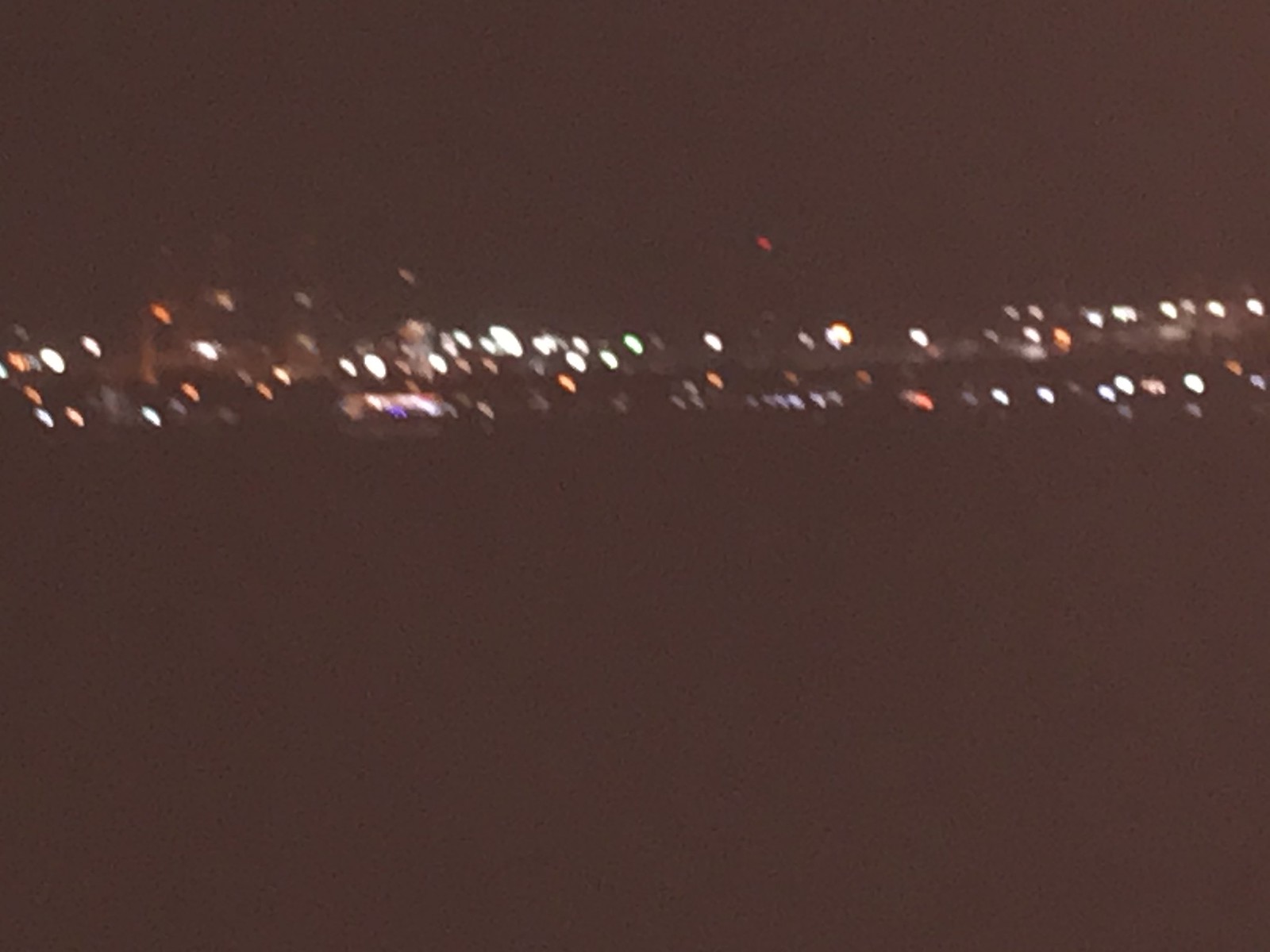This image presents a mysterious, blurry night scene characterized by an abundance of lights against a predominantly black background. Dominating the center of the image is an isolated red light, standing out starkly amidst a sea of glowing white and occasional orange lights. These lights create a trail that extends from the right side to the left side of the frame, suggesting the presence of a bridge or possibly a road running underneath it. On the left side of the image, there is a faint, almost indiscernible silhouette of a building, further obscured by fog or blur. This building is distinguishable by an orange light and a cluster of white lights, with a hint of pink intermingled. The scene conveys a sense of mystery and abstraction, where the exact details remain veiled by the pervasive blur and foggy atmosphere.